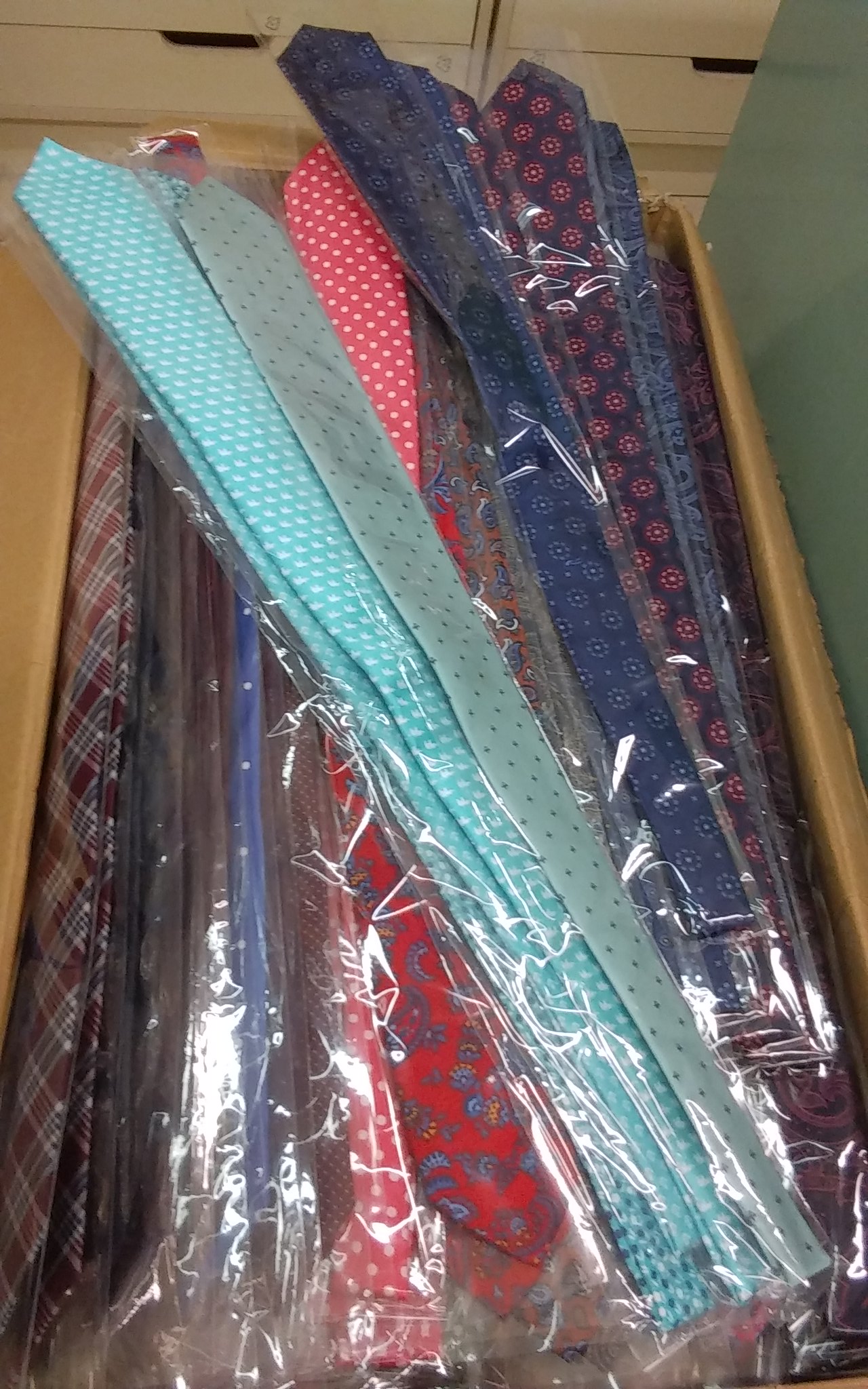The photograph shows a rectangular cardboard box filled with numerous ties that are individually wrapped in plastic. There are approximately 50 ties grouped in packages, each containing around three to five ties. The ties exhibit a variety of colors and patterns, including light blue ties with white spots, dark blue ties with floral designs, red ties with various motifs such as polka dots and stripes, and a distinctive flannel tie featuring red, blue, and white stripes. Also visible are ties with unique patterns like black with red flowers and dark purple with burgundy circles. In the background, the image shows white drawers with open notches and a light grayish-blue wall or cabinet, adding a subtle context to the overall setting.